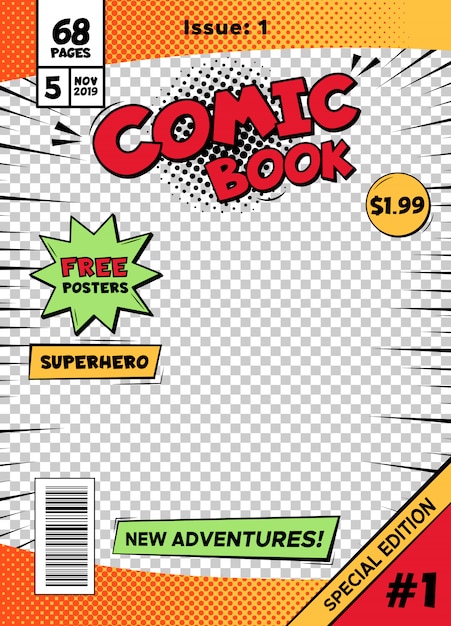This image is a vibrant, detailed template for a comic book cover, designed in a hand-drawn, comic-style font and art. At the top, in bold black text on an orange background, it clearly reads "Issue 1." Directly beneath this, in large red lettering with a black outline, the text "Comic Book" stands out prominently. To the left of this, a green starburst graphic exclaims "Free Posters Inside." Moving downwards, a yellow text box with black lettering declares "Superhero." Below this, near the barcode on the bottom-left corner, a green rectangular box advertises "New Adventures."

The central background area of the cover features a gray and white checkerboard pattern, mimicking a transparency texture typically used in design software. From the upper left corner, a white text box details "68 pages, 5, November 2019" in clear black text. To the right of the "Comic Book" title, the price is listed as "$1.99" inside a yellow circle. Finally, the bottom right-hand corner emphasizes "Special Edition Number One" in black text.

This cover is rich with classic comic book elements, including striking color contrasts, varied text styles, and dynamic graphic shapes, all set against a sophisticated, checkered backdrop.